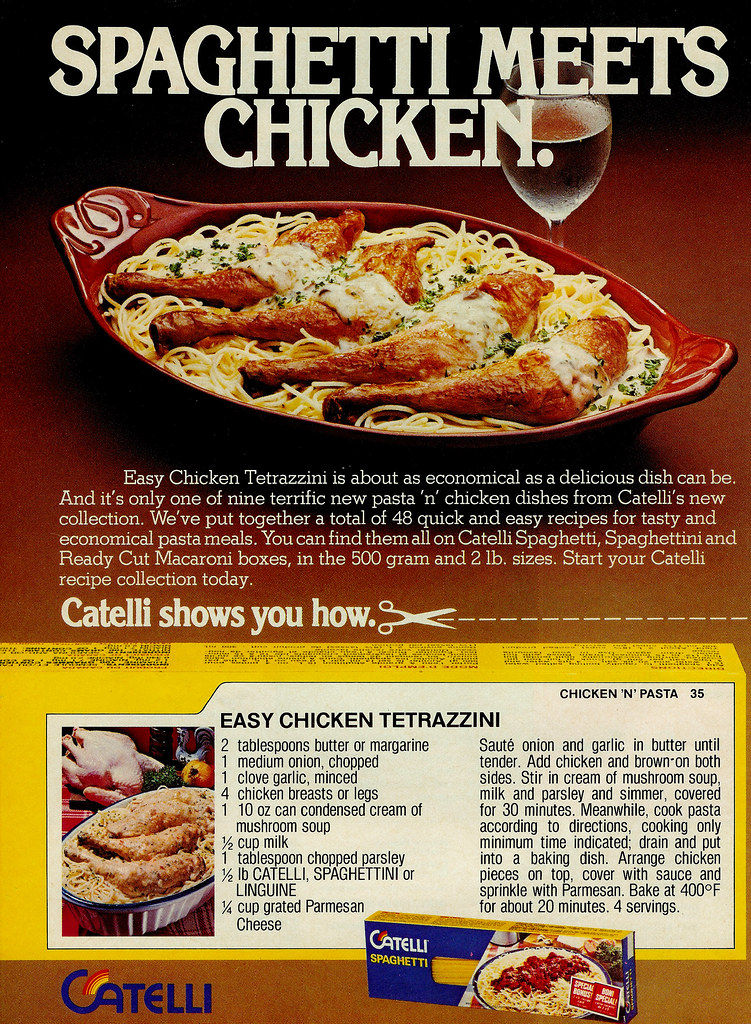The advertisement for Catelli's spaghetti features a vibrant red background with a prominently displayed bowl of spaghetti topped with chicken in a creamy white sauce, garnished with parsley. The headline reads, "Spaghetti meets chicken," emphasizing an easy chicken tetrazzini recipe that is both delicious and economical. The ad highlights that this recipe is part of Catelli's new collection of 48 quick and easy pasta dishes, designed to be affordable and tasty. The collection includes nine different pasta and chicken recipes, all of which are available on Catelli's product boxes, including spaghetti, spaghettini, and ready-cut macaroni in 500 grams and 2-pound sizes. The bowl of chicken tetrazzini is accompanied by a glass of wine, adding a touch of elegance to the meal presentation. At the bottom left corner, a box of Catelli spaghetti is displayed, with the brand name written in blue and featuring a distinctive half arch over the letter 'A' in colors red and yellow. The ad provides a detailed step-by-step recipe, making it accessible for anyone to recreate this flavorful dish at home. Start your Catelli recipe collection today and enjoy these easy and budget-friendly pasta meals.